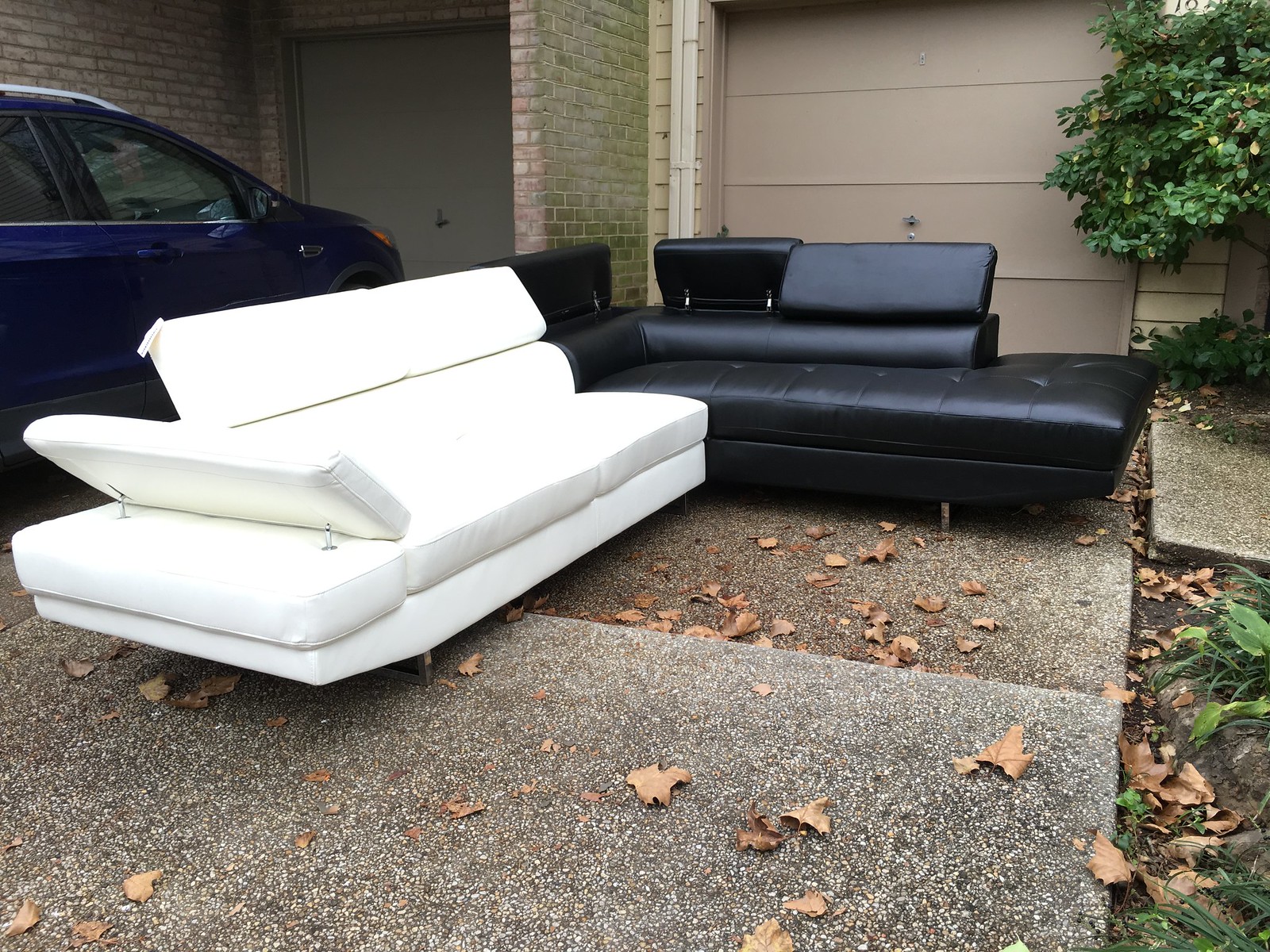This image captures a scene in a residential driveway with uneven concrete slabs scattered with dry, brown leaves. The focal point is an arrangement of two modern leather sofas. One black sofa, with an adjustable angled back and armrest, is positioned near a tan-painted garage door of a brick building. Perpendicular to it is an identical white sofa on gold metal legs, extending from the center left to the lower right of the image. The house, constructed from beige and reddish brick, features a double garage, with a dark blue or black vehicle, possibly an SUV or van, partially visible in front of the left garage door. To the right, a narrow sidewalk lines the edge of the driveway near a small tree, enhancing the quaint, residential atmosphere of the overcast scene, illuminated by soft, diffused light.